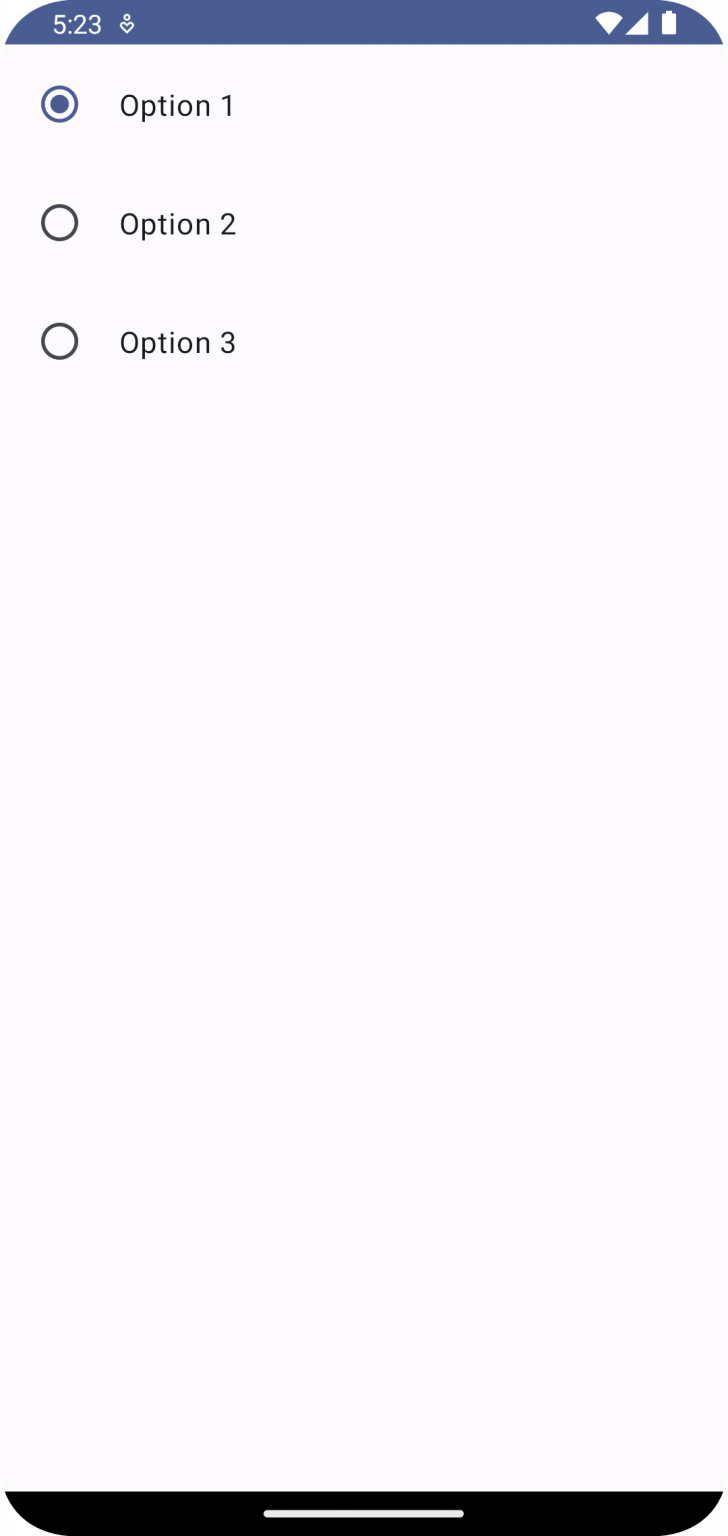The image appears to be a screenshot taken on a phone. The background is primarily a dark bluish color. At the top right corner, there are three status icons: a vertically-oriented white battery icon, a fully covered white phone signal strength icon, and a fully covered white Wi-Fi icon. On the top left, the time is displayed in white as "5:23", next to which sits a small icon resembling a heart-shaped body with a circular head.

Directly below this top section, there are three selection bubbles. The first bubble, labeled "Option 1", is blue and checked, indicating it is selected. The subsequent two bubbles, labeled "Option 2" and "Option 3", are black and unselected. This section has a grayish background. 

At the very bottom of the screenshot, there is a white rectangular home bar.